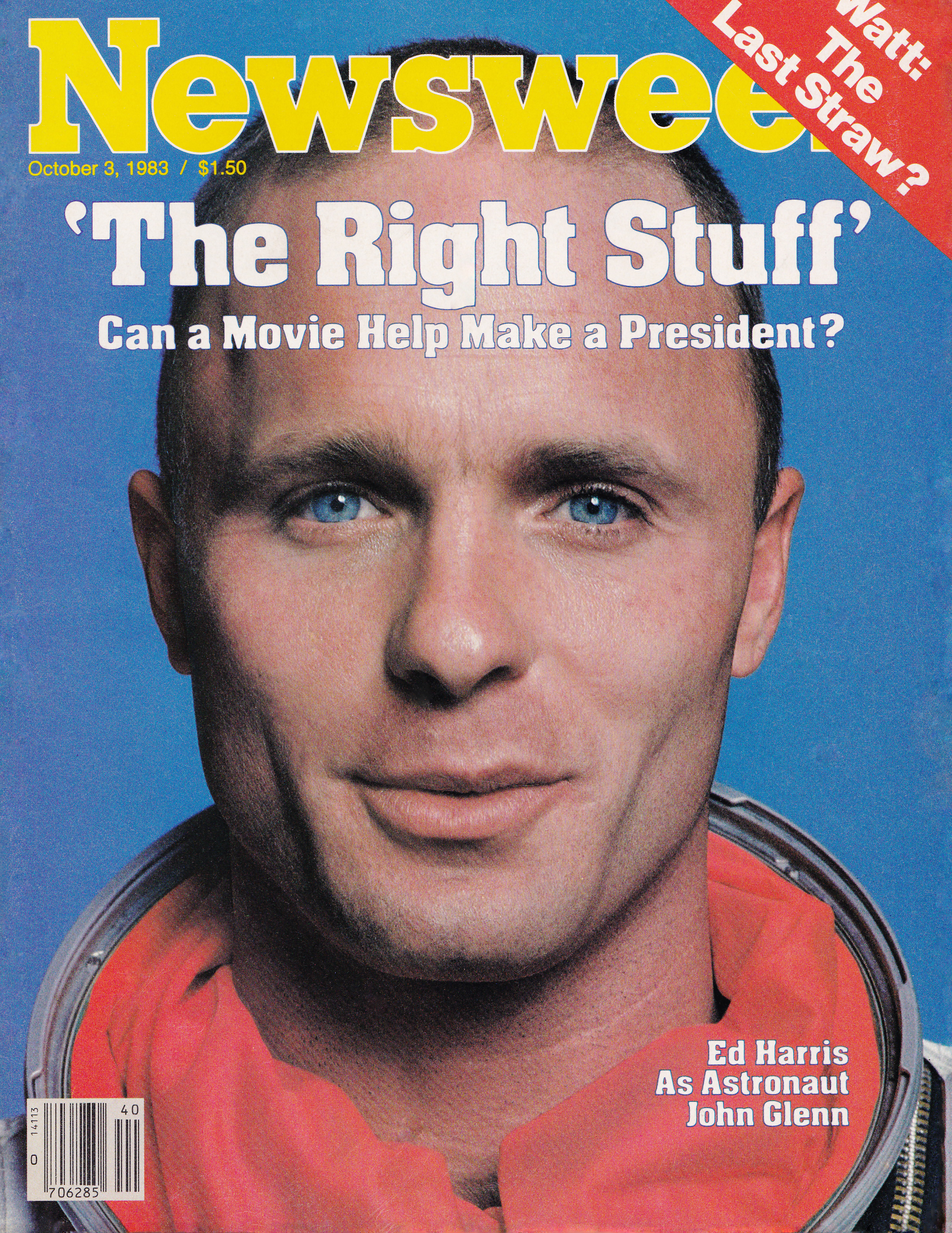The magazine cover of Newsweek dated October 3rd, 1983, priced at $1.50, features a young Ed Harris as astronaut John Glenn. The background is blue, and the top banner in yellow reads "Newsweek." Dominating the cover, Ed Harris is depicted with short, light brown hair and striking blue eyes in a helmet-less astronaut suit. Overlapping his image, the bold text reads, “The Right Stuff: Can a Movie Help Make a President?” In the upper right corner, within a red triangular banner, is the intriguing headline, "Watt: The Last Straw?" The bottom left corner houses a black-and-white barcode, completing the detailed layout of this iconic magazine cover.